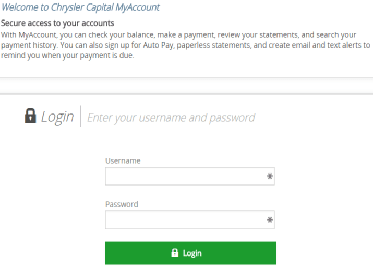The image is a screenshot of a login page for Chrysler Capital's "My Account" portal, set against an all-white background. At the top left corner, the text "Welcome to Chrysler Capital, My Account" is displayed in bluish-green lettering. Directly below this, in black text, it reads "Secure Access to Your Accounts." The purpose of the portal is clearly outlined, stating you can check your balance, make payments, review statements, and search payment history. It also notes options for signing up for AutoPay, paperless statements, and setting up email and text alerts for payment reminders.

Below this information, two horizontal gray lines provide separation. Just under the last gray line, on the left side, there is a black padlock icon. To the right of the padlock, in gray text, it reads "Log In | Enter Your Username and Password." Two text fields follow: the first for "Username," labeled in black, is empty with a black dot or arrow on its right side (the detail is slightly blurry). The second text field, labeled "Password" in black, is similarly empty and also features a black dot or arrow on the right side.

Below these fields, there is a wide emerald green button with white text that says "Log In." To the left of the "Log In" text, a white padlock icon is displayed, symbolizing security.